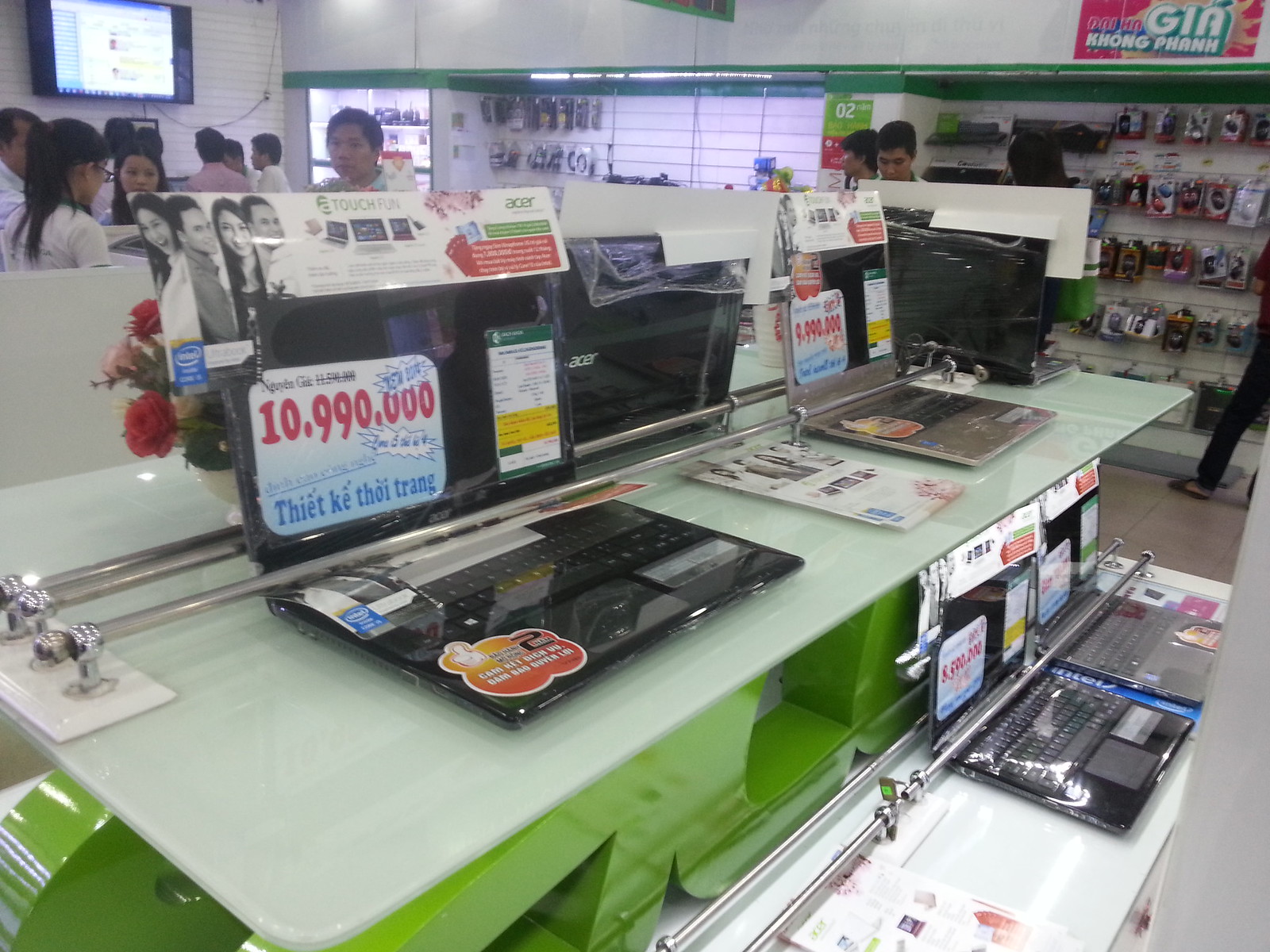This image depicts a bustling electronics store in Vietnam, evidenced by the Vietnamese language on the signage. At the forefront, several Acer laptops are showcased on a white countertop table with a lime green base. One of the prominently featured laptops is listed at 10,990,000 VND, roughly equivalent to $400-$500 USD. To prevent theft, a metal rod runs across the middle of the laptops. The store layout includes two shelves displaying various tech gadgets, and to the right, the wall is adorned with packaged items like headphones, speakers, and computer mice. On the left side, customers can be seen browsing, and at the back corner, a television is mounted on the wall. Multiple signs and descriptions highlight the prices and features of the products. The lively atmosphere and organized security measures reflect a well-maintained retail space.